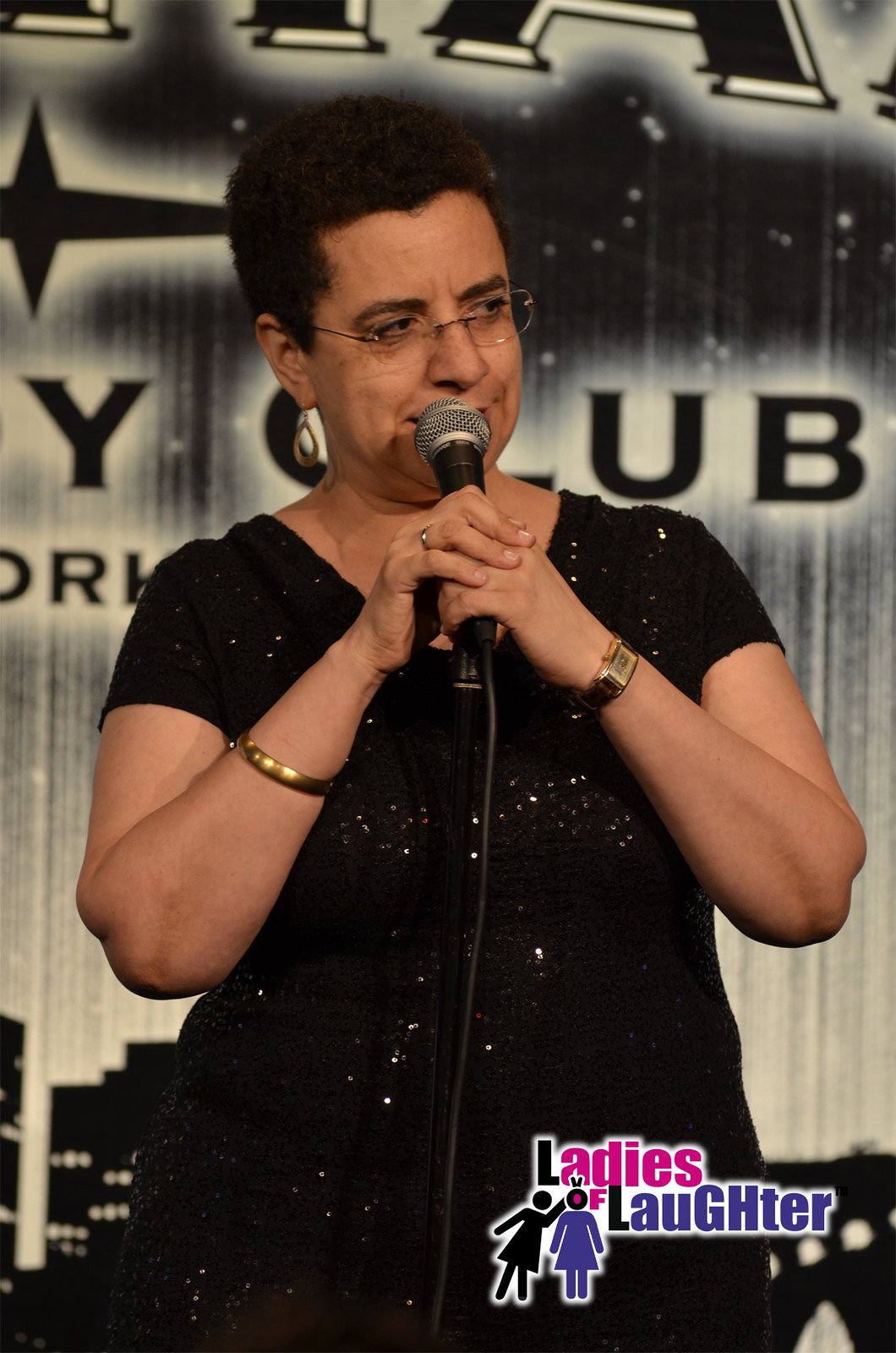The image captures a woman standing on a stage, holding a black microphone with a silver top close to her mouth, partially obscuring her lips. She has short black or dark brown hair, which appears to be pulled back into a ponytail, and is wearing eyeglasses. Her expression is sharp, suggesting disapproval. She dons a black outfit, which might be a short-sleeved blouse with dots in red, green, and white, paired with black pants. A gold bracelet adorns her left arm, while her right wrist sports a black-faced watch with a black band. She also wears a ring on her left hand and big gold earrings. The background features a gray and white backdrop with partial text, including visible letters like Y, U, and B. Some elements of a cityscape are faintly discernible. The text "Ladies of Laughter" appears in the bottom right corner, with "Ladies" in pink (except for the black 'L') and "Laughter" in purple (except for the black 'L'). The logo features two stick-figure women silhouettes: one black, leaning over with a peace sign over the head of the other, which is purple with a black head and a central red dot.